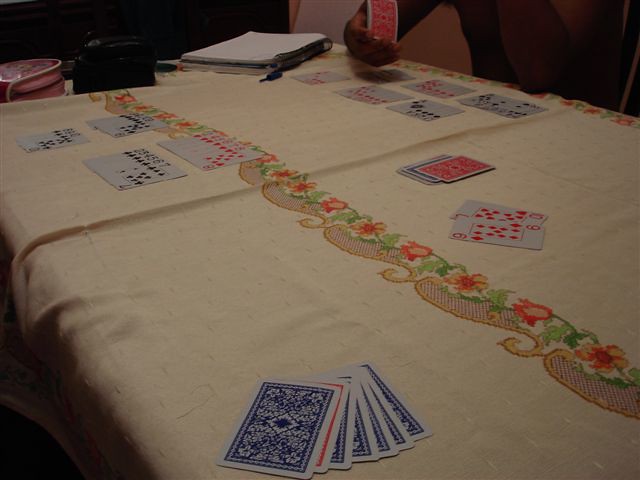The image portrays an intense card game in progress, set on a table adorned with a simple tablecloth. The focus of the scene centers around a diverse array of playing cards arranged meticulously for a two-player game. One player's hand, brown-skinned and poised, holds a card with a striking red back, hinting at strategic moves. The table itself is a vibrant mix of red and blue-backed cards, interspersing the competition. To the left and right of the scene, cards are grouped by suit in organized sets of four for each player, suggesting structured gameplay. Close to the visible player's hand, a spiral notebook and a pen cap lie casually, possibly for noting down scores or strategies. In the far bottom center, a distinct set of seven cards lies face down, slightly fanned out, predominantly blue with a solitary red-backed card second in the sequence. An additional pile of cards features two face-up cards atop a mix of face-down reds and blues, further indicating the game's dynamic progression.